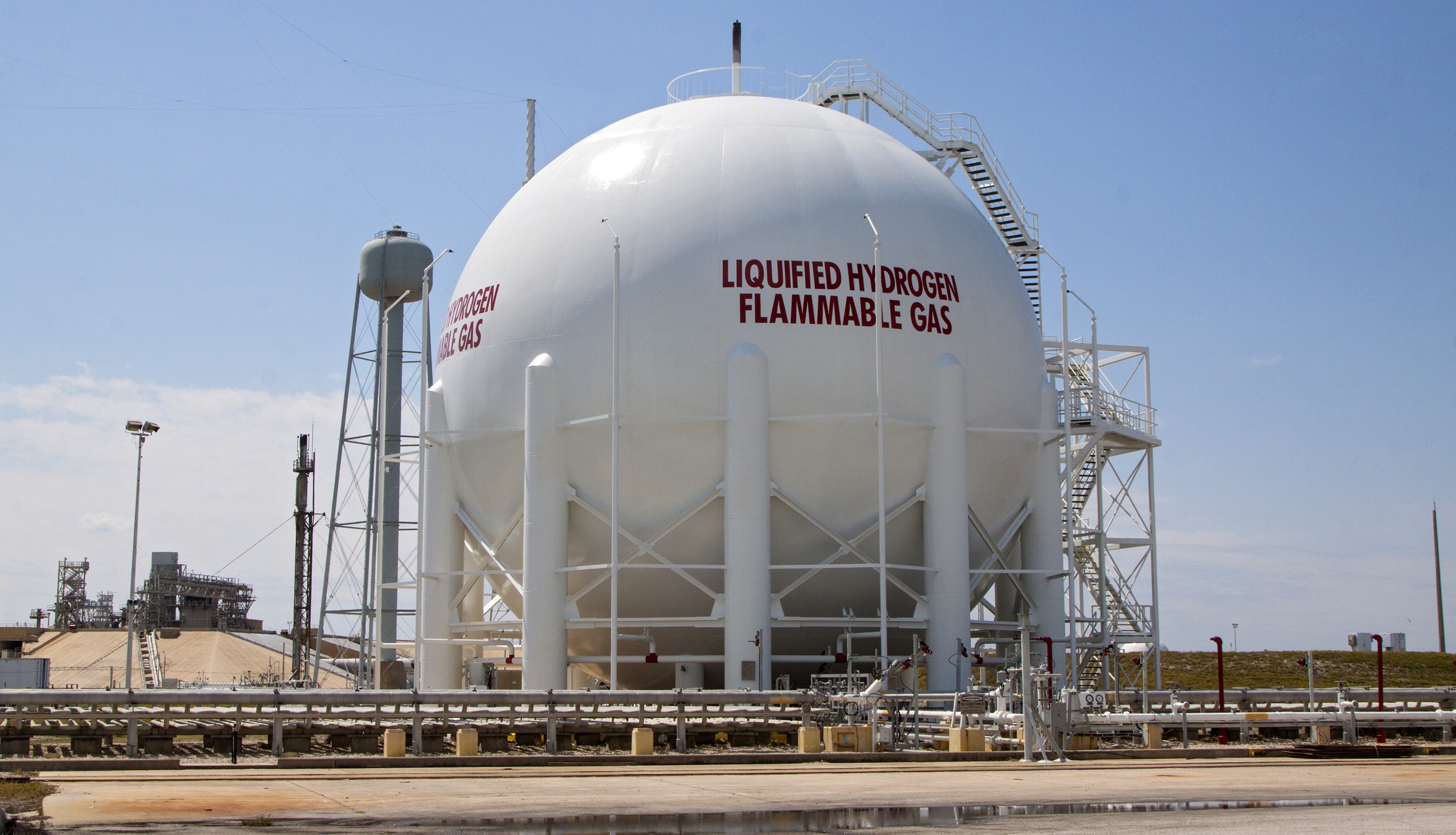The image showcases a large, spherical white tank labeled "Liquefied Hydrogen Flammable Gas" in red letters. The tank, resembling a massive ball, stands prominent with multiple staircases on its right side, indicating its immense scale. It is supported by white legs that extend to the ground, resembling interlocking girders. Surrounding the tank is a small fence and railings that maintain safety and restrict access. A smaller, gray tower, resembling a water tank with a long pipe, is positioned behind the main structure. The scene is set against a bright blue sky with a hint of clouds on the left, typical of an outdoor industrial area. A road runs in front of the facility, and additional machinery is visible in the lower left part of the background, further detailing the gas refinery environment.